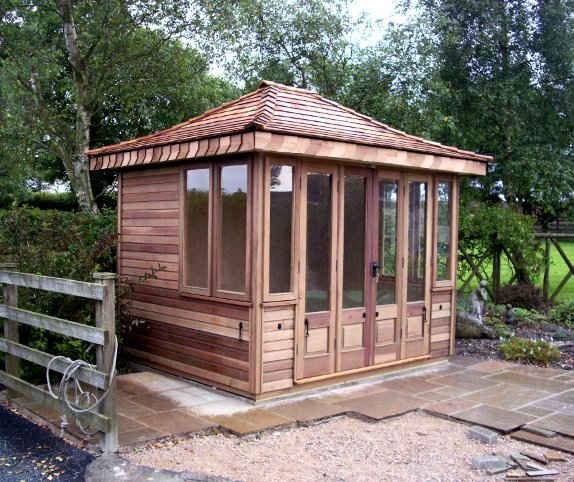The image captures a detailed scene of a small outdoor wood-structured building, or gazebo, positioned prominently in the center. Set against a backdrop of towering trees with lush green leaves and glimpses of a bright daytime sky, the gazebo stands on a tiled stone pathway, partially covered with gravel indicating ongoing construction. The gazebo, crafted from horizontal wood slats in varying shades of dark and light brown, features a four-sided wood tiled roof. The front façade is adorned with five long, narrow windows, two of which are part of the entry doors, though it’s unclear if the doors are single or double. The building’s left side reveals two slightly wider narrow windows on the corner. Surrounding the gazebo is a wooden fence, visible to the left and comprising four horizontal slats with a rope near the bottom. The color palette of the image includes natural tones of brown, green, gray, and white, highlighting the earthy outdoor setting, potentially someone's yard or an outdoor barbecue area.